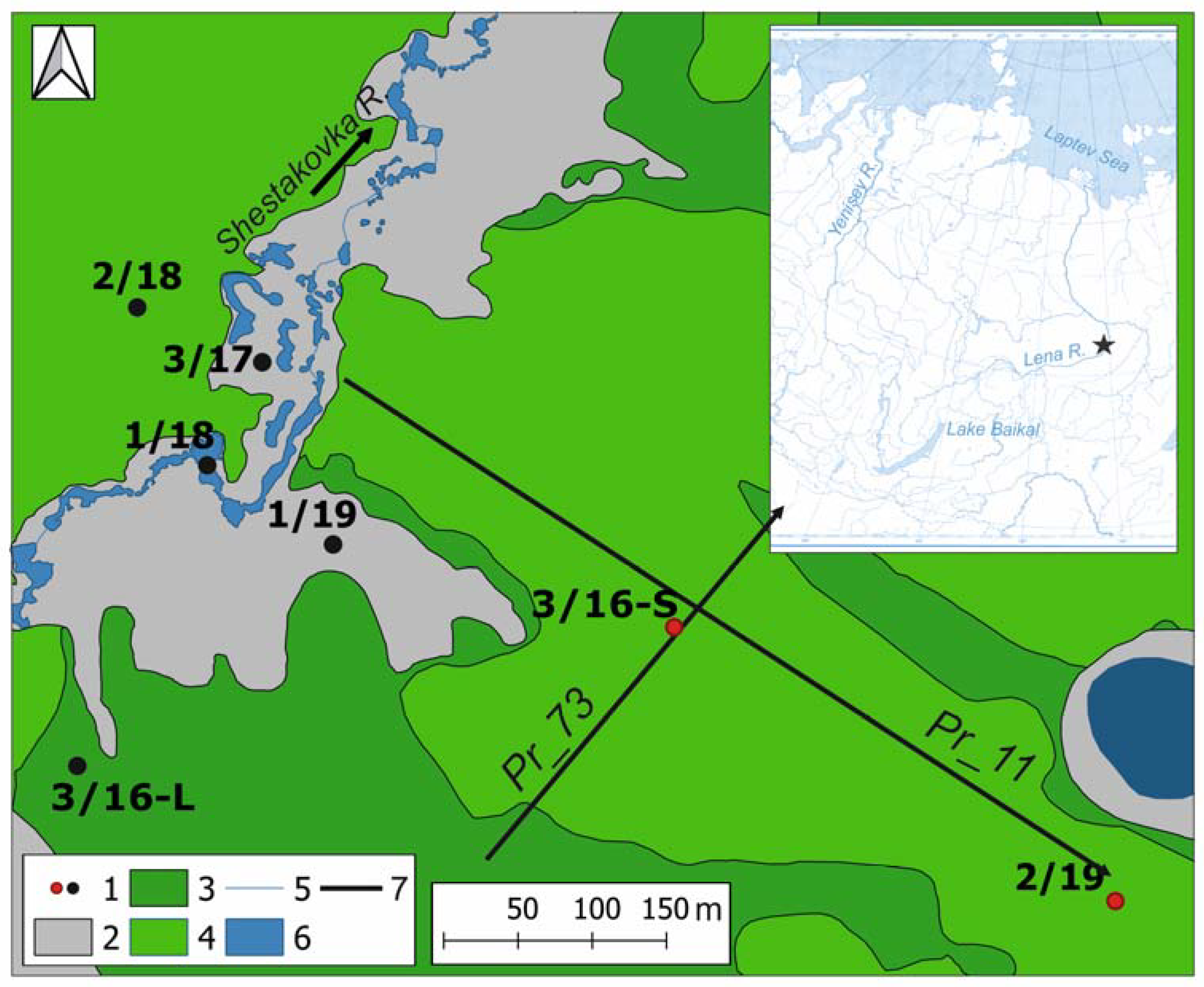The image, shaped as a horizontal rectangle, depicts two maps: a main map in light and dark green hues, and a smaller, zoomed-out map in the top right, rendered in white and blue. Both maps appear to be digitally created, featuring precise lines and clear colors. The central, larger map showcases various shades of green to indicate different elevations, with darker green patches at the bottom, top, and far right. Water bodies on this map are marked in blue and grey, with the grey splotch located in the top left. Black text on this map includes the word “Shestakovka” accompanied by a black arrow.

The smaller map in the top right appears superimposed and outlines four notable places in blue text: Lake Baikal in the south, the Laptev Sea in the north, the Yenisei River in the west, and the Lena River in the center, marked with a star. This inset map contrasts with the main map’s green tones by using white to represent land and blue for water. Additionally, the image contains a key at the bottom that provides a scale of 150 meters and lists color-coded references: 1 (black and red dot), 3 (green), 5 (grey line), 7 (dark line), and another key with 2 (grey box), 4 (light green), and 6 (blue).

In summary, this detailed visualization combines a primary, more detailed green map with a supplementary, broader white-and-blue map inset, each providing valuable geographic and topographic information through distinct legends and labels.